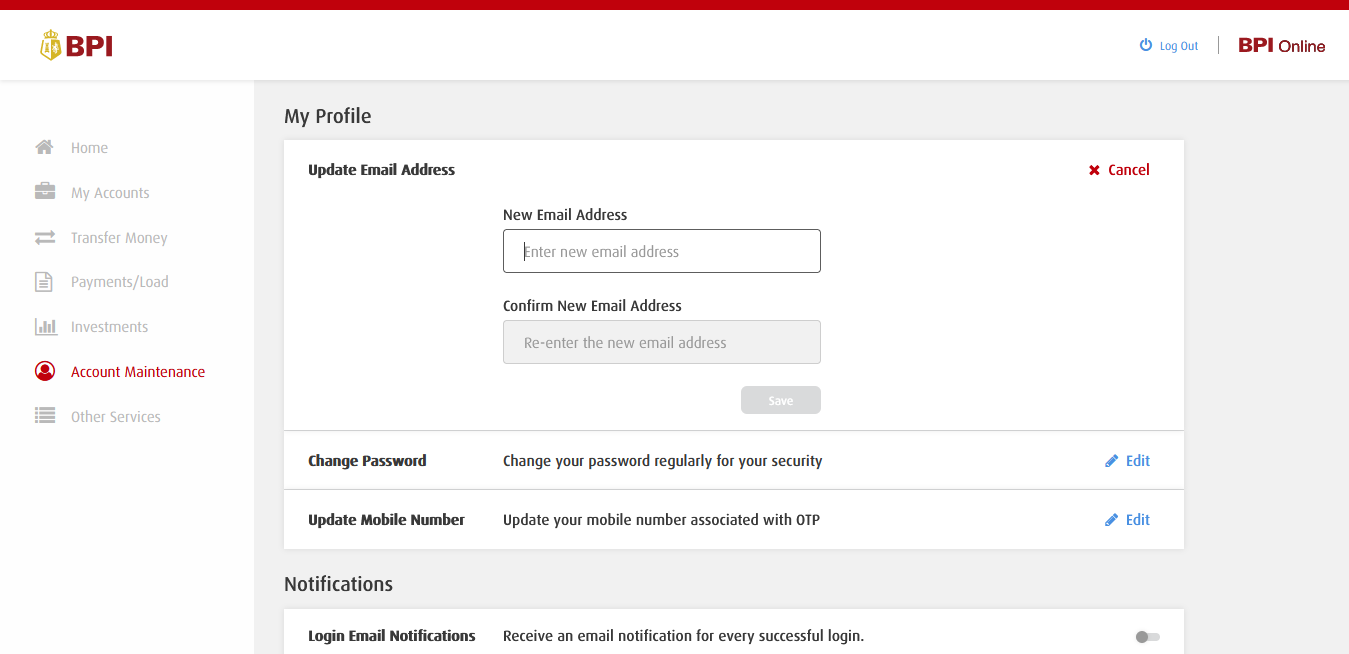The screenshot depicts a user interface of a website or an app, displayed on a computer screen. The top of the screenshot features a prominent horizontal red line. Below this line, on the left side, there is an almost indistinct yellow-gold logo, adjacent to the letters "BPI" written in bold, red capital letters. On the right side of this red line is a "Log out" option in blue ink, and "BPI online" also written in dark red ink.

Further down, there is a menu bar with several options organized horizontally. These options include "Home," "My Accounts," "Transfer Money," "Payments," "Loads," "Investment," "Accounts Maintenance," and "Other Services," each accompanied by an icon. The text for these options is grey, with the exception of "Accounts Maintenance," which is highlighted in red to indicate it is the current selection.

On the main screen, the user’s profile section is shown with the title "Update Email Address" displayed prominently. There is a "Cancel" button in red and an "Edit" button in blue, while the remaining text is in black.

Overall, the layout is clean and organized, using a color scheme of red, blue, grey, and black to differentiate between various elements and functions.